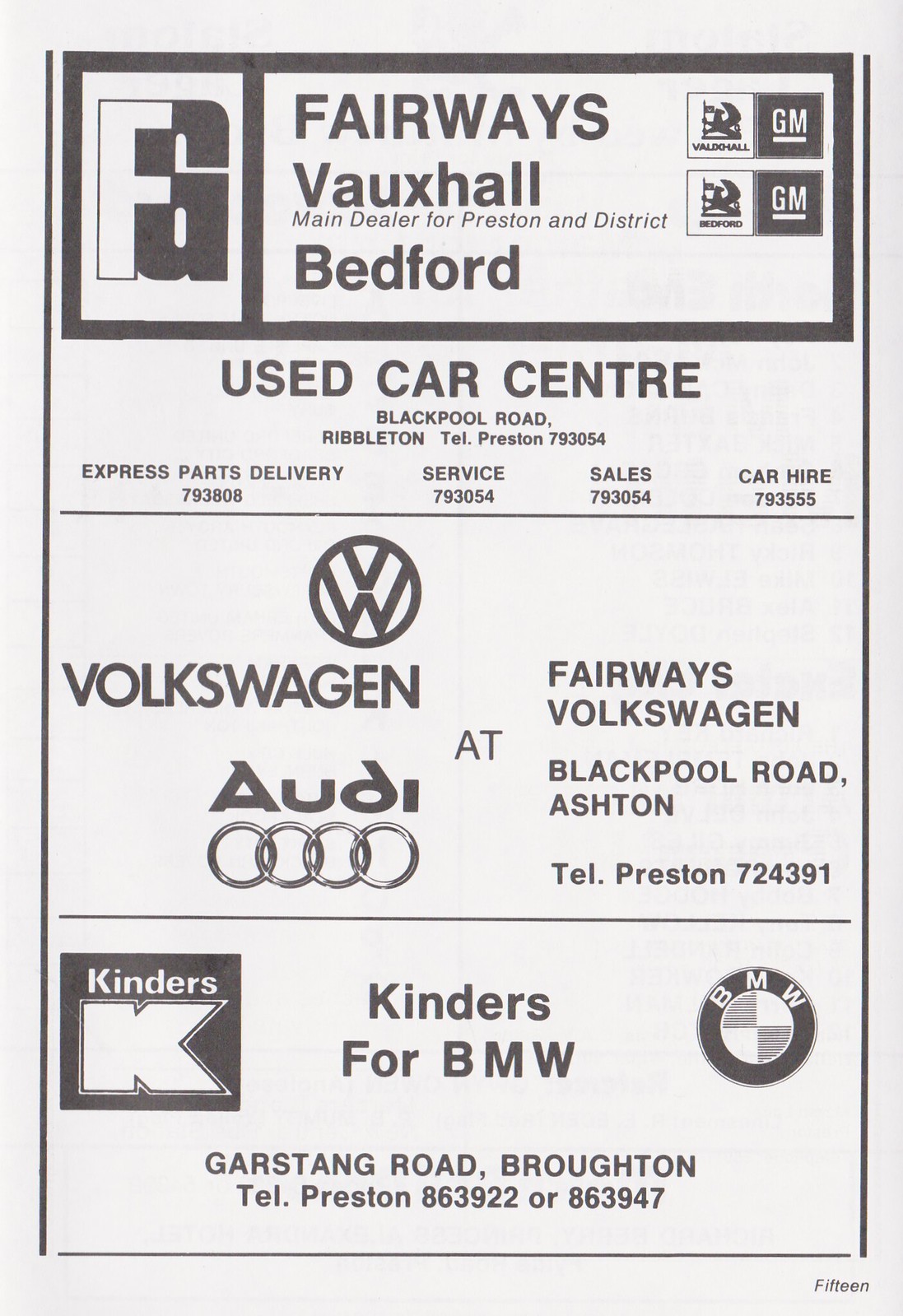The image is an advertisement printed on old, beige paper with black text and features a prominent, thick black border at the top. Positioned centrally, the advertisement details various automotive services and dealerships. At the very top in a small, square box on the left-hand side, the letters "F" and "G" are displayed. The main headline reads "Fairways, Vauxhall GM, Bedford GM, Used Car Center," emphasizing their role as a main dealer for Preston and surrounding districts. Below, it highlights services offered, including parts delivery, service, sales, and car hire, with specific sections for Volkswagen and Audi dealerships located on Blackpool Road, Ribbenton. The advertisement also provides multiple telephone numbers for different services, with repeated listings for "Fairways, Volkswagen at Blackpool Road, Ashton," and "Telephone Preston 793054" and other specific contact numbers for different services. The bottom right-hand corner of the ad features the number "15" spelled out.